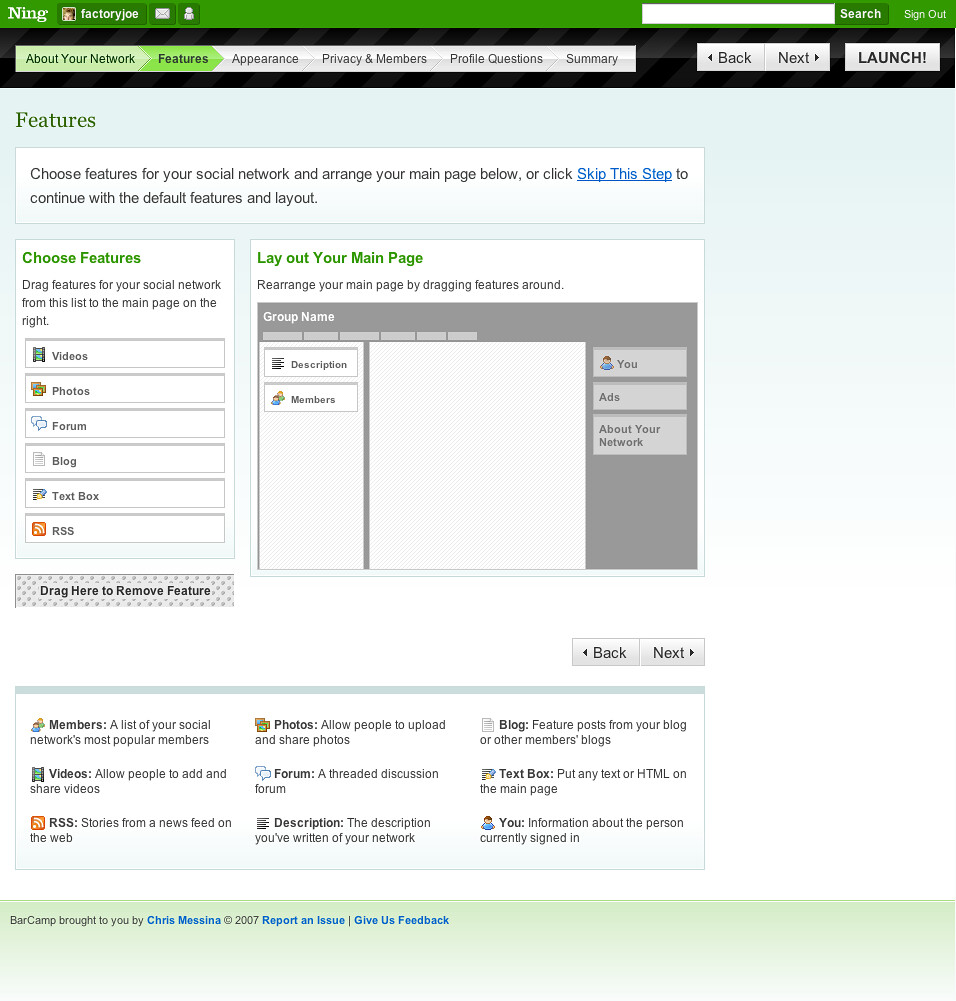This image is a screenshot of a user's account page from Ning, a now-defunct social networking site. The page features a distinctive green top border, with the word "Ning" prominently displayed in white on the upper left corner. The user's username-- which appears to be Factory Joe, though the font is small and difficult to read-- is also visible. 

An avatar next to the username is present but too small to discern any details, appearing as a light brown icon. On the right side of the top border is a rectangular white search box. Below this, a navigational menu on a silver-gray background is displayed, with options labeled from left to right as: About, Your Network, and Features (this option is highlighted in green), followed by Appearance, Privacy and Members, Profile Questions, and Summary. 

On the far right, there are three silver-gray rectangular buttons labeled Back, Next, and Launch. Directly beneath this, against a very light blue background, is a white box titled "Features." This section provides an instruction: "Choose Features for Your Social Network, and Arrange Your Main Page Below," with an option to "Skip This Step," highlighted in blue and underlined, allowing the user to proceed with default features and layout.

The page offers customization options, with a left-hand sidebar under the header "Choose Features," and a larger box on the right labeled "Layout Your Main Page." At the bottom, there is a glossary explaining terms related to the customization options, organized into three columns.